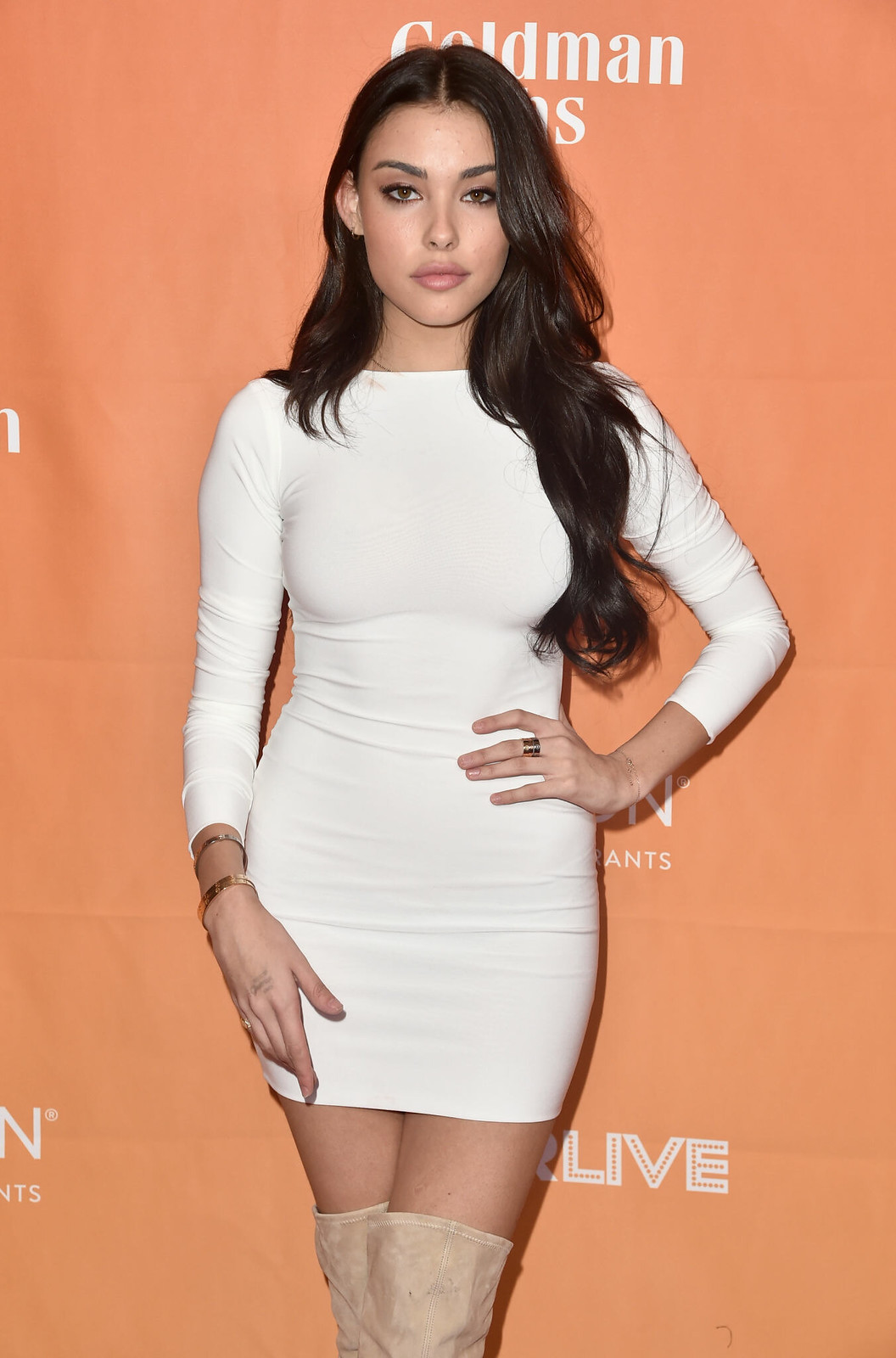The photograph captures a professional red carpet moment featuring a young woman, possibly Madison Beer, standing against an orange banner adorned with partial logos including "Goldman Sachs" and "LIVE." The woman, showcasing a poised and serious demeanor, has long dark brown hair cascading down her chest on the left side, partially revealing her ear on the right. She is attired in a form-fitting, long-sleeve white mini dress enhancing her elegant silhouette. The dress reaches her forearms and is complemented by beige over-the-knee boots, leaving a sliver of skin visible between the hem of her dress and the tops of her boots. She accessorizes with bracelets on her right wrist and a ring on her left middle finger. The woman is striking a confident pose with her left hand on her left hip and looking directly at the camera, projecting an aura of sophistication amidst the event's backdrop.